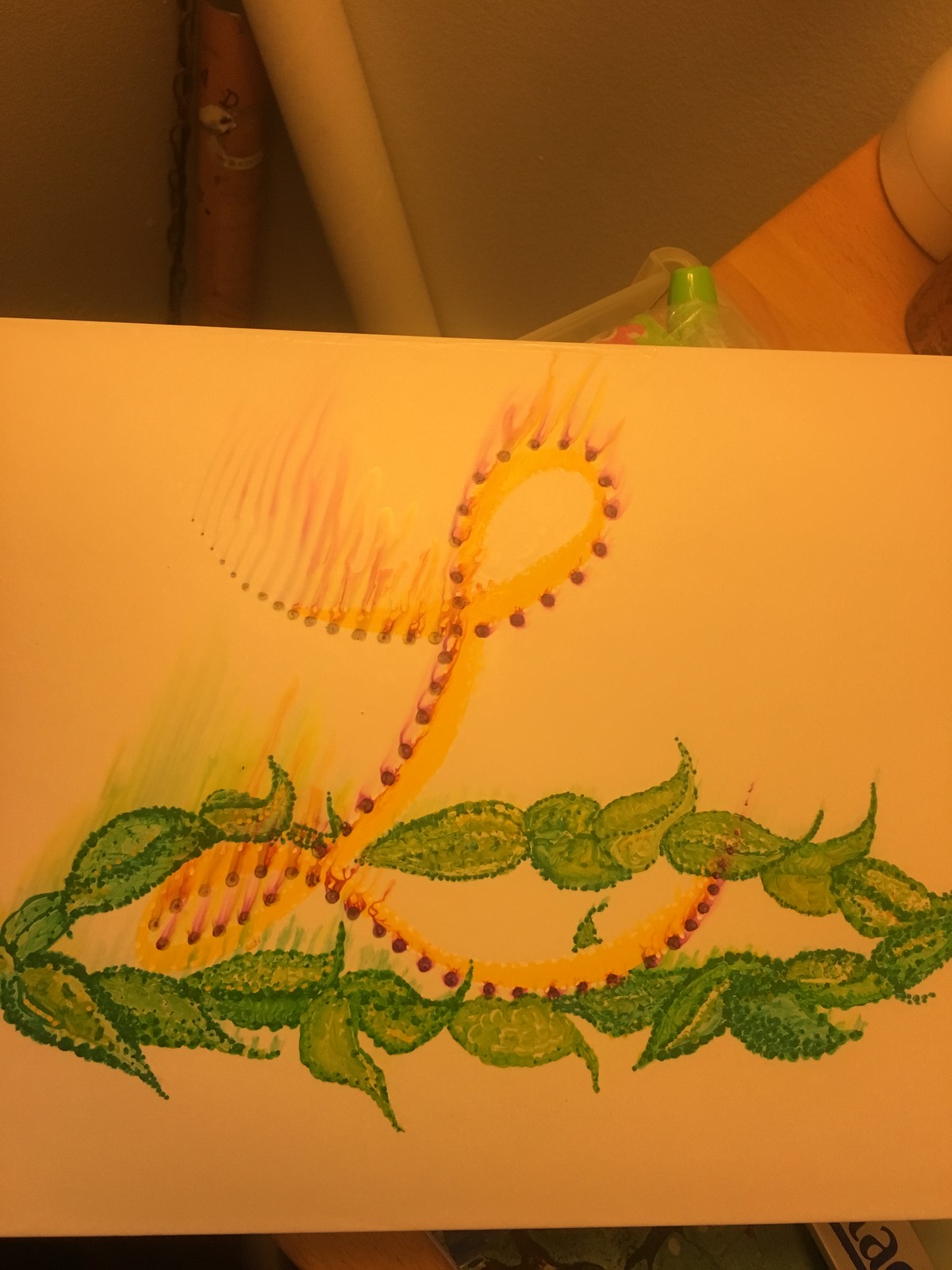The image depicts an intricately detailed sketch that appears to be created using colored pens. Predominantly done in pen, the medium slightly bleeds, lending it a soft, blended appearance. At the centerpiece of the artwork is a laurel wreath, reminiscent of Roman crowns. The wreath, composed of green leaves, encircles the bottom of the page, with each leaf meticulously outlined in darker dots and then lightly filled in with color for a dimensional effect. 

The wreath forms a complete circle, symbolically positioned to convey strength and victory. Just above the midpoint on the right side, where the leaves converge, is a striking cursive "L" rendered in red ink. This letter ascends gracefully towards the top of the page and then descends, with its lower curve weaving through the leaves and extending downwards. Some sections of the red ink exhibit a subtle yellow hue, suggestively bleeding upward, which might be an intentional artistic choice or an artifact of the medium.